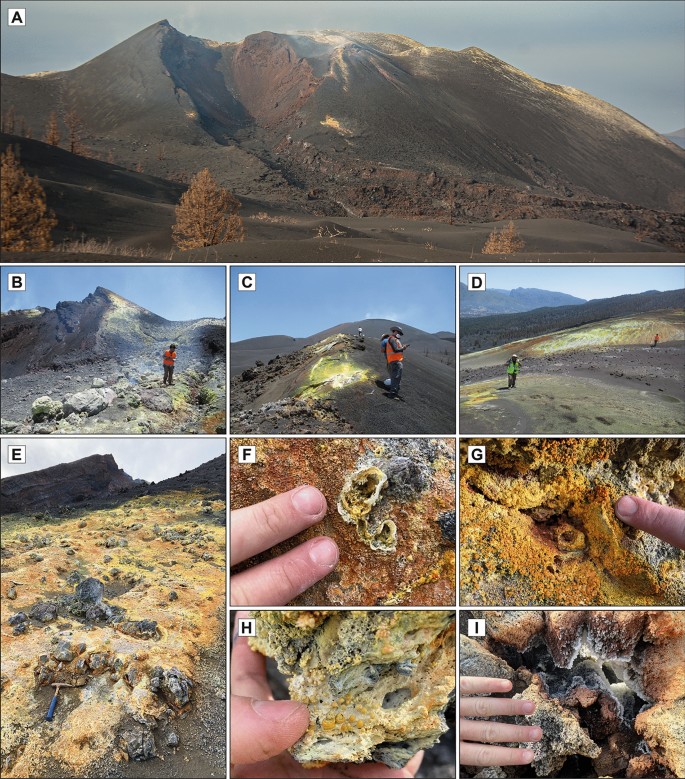This image features a 3x3 grid of nine photographs labeled A through I, capturing various aspects of a mountainous landscape and geological details. 

1. **Image A**: A wide landscape photo depicting a dark, brown mountain with a few trees in the foreground. The mountain is slightly snow-capped, and the sky is a blend of blue with some white clouds.
2. **Image B**: A closer view of the mountain terrain showcasing a person wearing a red or orange vest, standing amidst the rocks.
3. **Image C**: A small hill at the base of the mountain, featuring two people in the frame. The sky remains clear and blue.
4. **Image D**: A closer section of the mountain terrain, again showing a person whose details are hard to discern.
5. **Image E**: A relatively wider shot, focusing on a rocky terrain with a hammer visible, indicating some geologic activity or fieldwork.
6. **Images F, G, H, and I**: These are close-up shots highlighting the texture and composition of the rocks. Fingers and hands are pointing at specific features, showing detailed, caked-on, yellowish-orange discoloration and possibly rust-like textures on the rocks.

The images collectively provide a detailed look at the mountainous area, the human presence and activity, and the close-up geological features of the terrain.